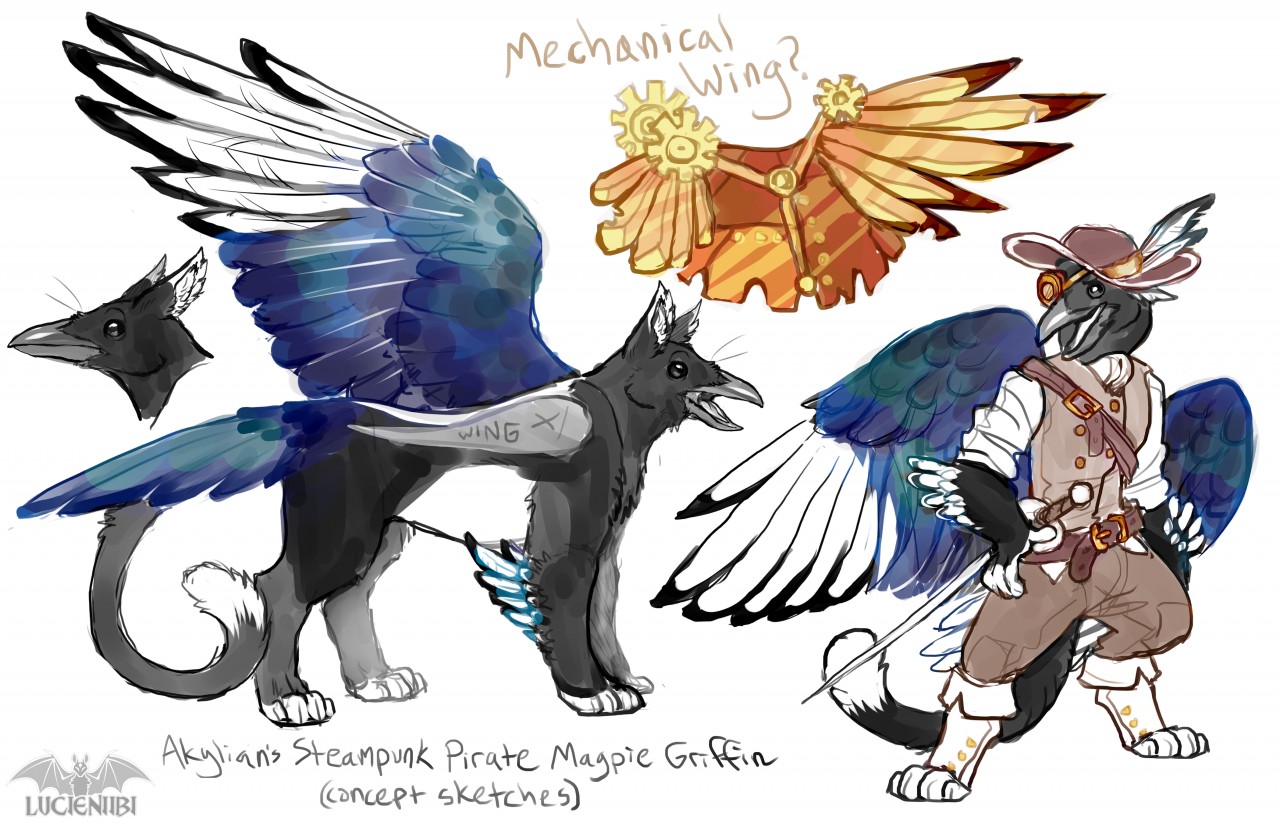This whimsical page from Lucienne E.B.'s sketchbook, signed in gray letters with a gray bat perched above the signature, is a detailed exploration of Steampunk Pirate Magpie Griffin concept sketches. Dominating the page is a fantastical griffin, featuring a beaked head, resembling a crow, with dog-like ears and the body of a cat. The unique creature boasts striking wings in various shades of blue with white wingtips. Nearby, there is a smaller sketch of the griffin’s head.

Above these sketches, the words “Mechanical Wing?” are prominently featured alongside a detailed drawing of an orange and brown mechanized wing, adorned with gears and designed in earthy tones. This adds an additional layer of whimsy and fantasy to the composition.

In the bottom right-hand corner, the griffin reappears in full steampunk pirate regalia. Dressed in pirate boots and a costume reminiscent of the Three Musketeers, featuring a feathered hat, the griffin strikes a pose that evokes a daring swashbuckler. The character also sports a steampunk eye patch, enhancing its adventurous appearance. This richly detailed page embodies a blend of fantasy, steampunk aesthetics, and imaginative character design.